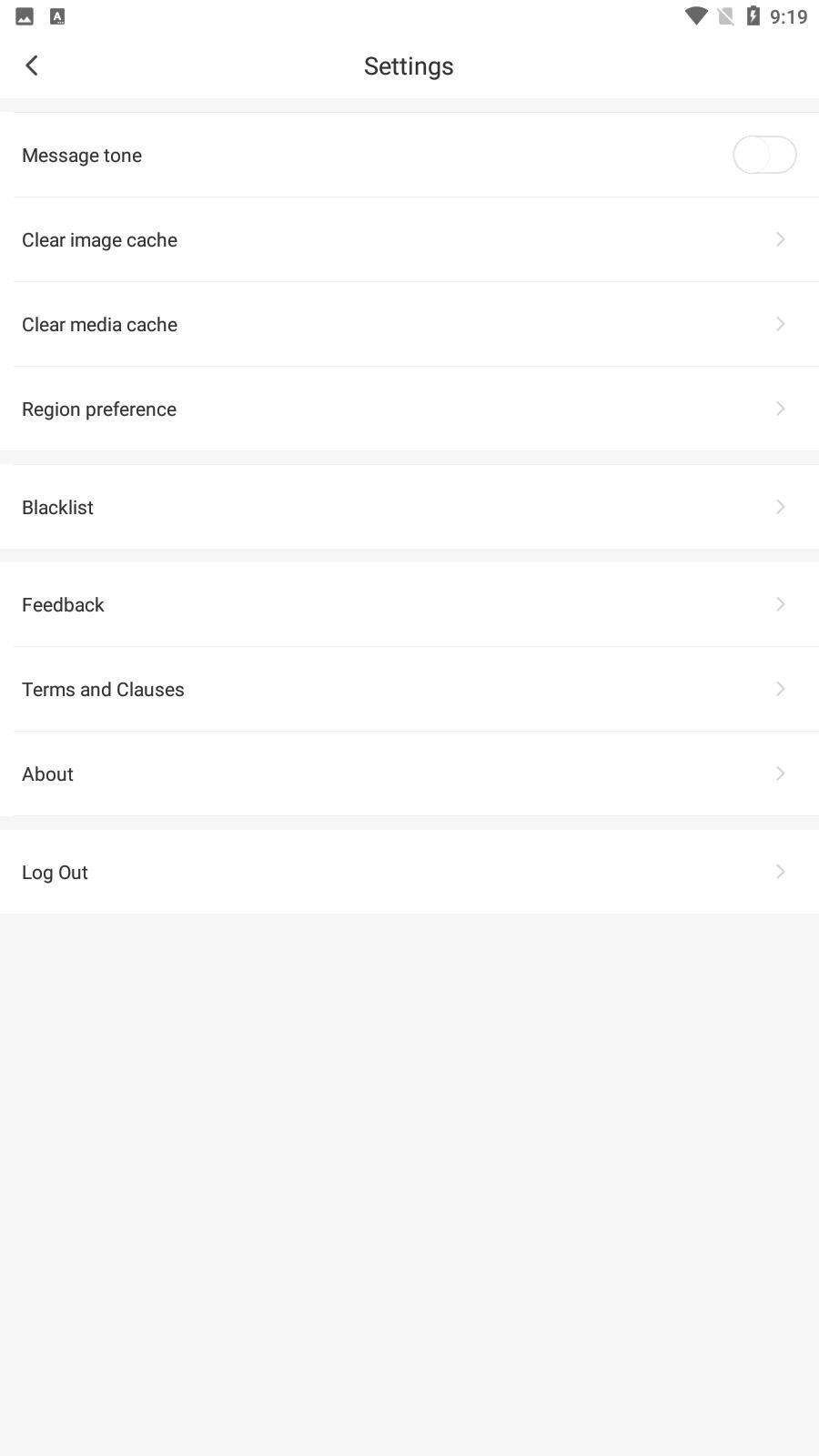A detailed portrayal of the user interface of a mobile device screen is depicted against a white background. In the top left corner, there is a gray square featuring a white mountain icon, signifying an image or photo. Adjacent to it, a green square with a white letter "A" displays. To the right, a gray Wi-Fi signal icon is present. Additionally, a box with a line through it, whose meaning is unclear, is visible. 

Further right, a battery icon stands out in gray with a white lightning bolt inside it, indicating that the battery is currently charging. Beside the battery, the time is shown as 9:19 in gray text.

On the subsequent row, there is a gray arrow pointing to the left, followed by black text that reads "Message Tone" on a white background. Below this, a section header with a gray border displays options including "Clear Image Cache," "Clear Media Cache," "Region Preference," and "Blacklist," each starting with a capital letter.

The screen continues with further options such as "Feedback," "Terms and Conditions," "About," and finally, "Log Out." Each of these items is prefixed by a gray border and uses capital letters for their initial characters.